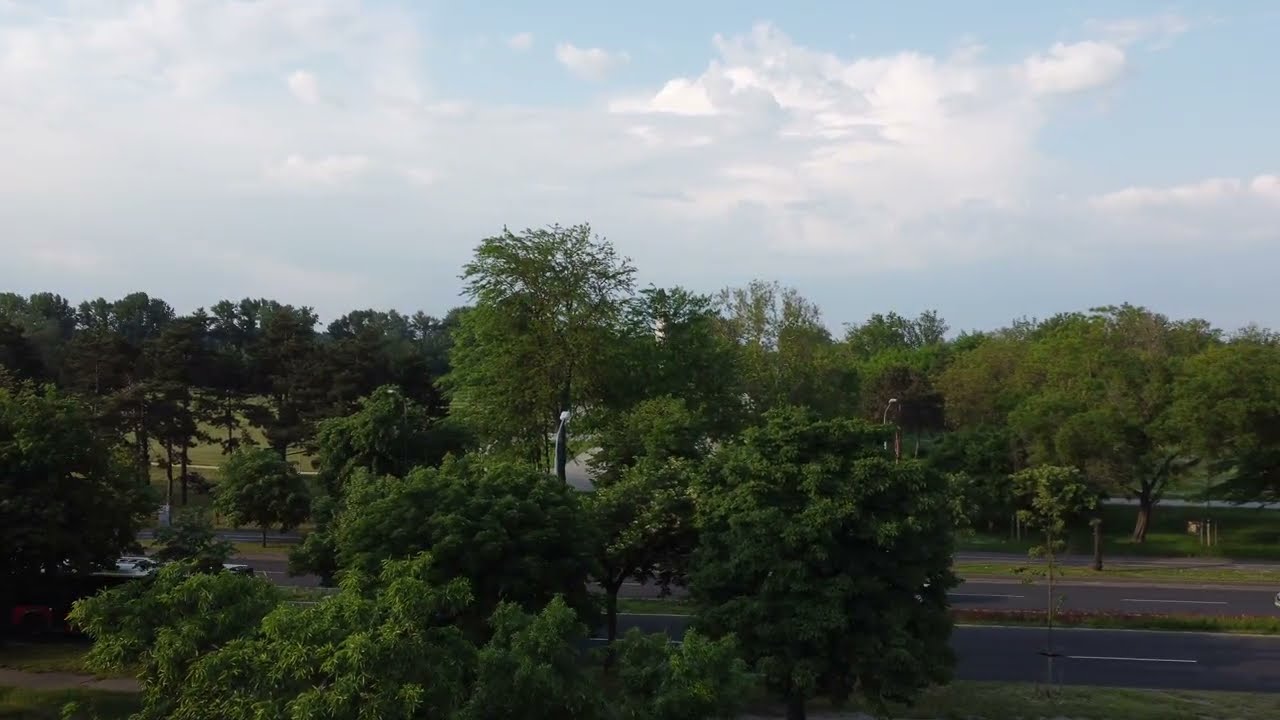The image depicts a vibrant outdoor scene dominated by a dense cluster of green trees, particularly prominent in the front center and extending into the background. The trees vary in height and shades of green, with some appearing tall and majestic. Beyond the trees, a four-lane, dark paved highway runs horizontally through the scene, partially obscured by the foliage. On the left-hand side of the highway, a few white cars are visible. The road features a grassy median dividing the lanes, which adds to the greenery. In the background, a glimpse of possibly a golf course or a small river/lake can be seen, adding to the complexity and natural beauty of the scene. The sky above is mostly clear with puffier white clouds scattered across a blue backdrop. The lush green trees, the dark highway, and the white clouds create a striking palette of colors, with hints of grays, browns, and pale yellow interspersed. Streetlights line the highway, adding a subtle human element to this predominantly natural landscape.